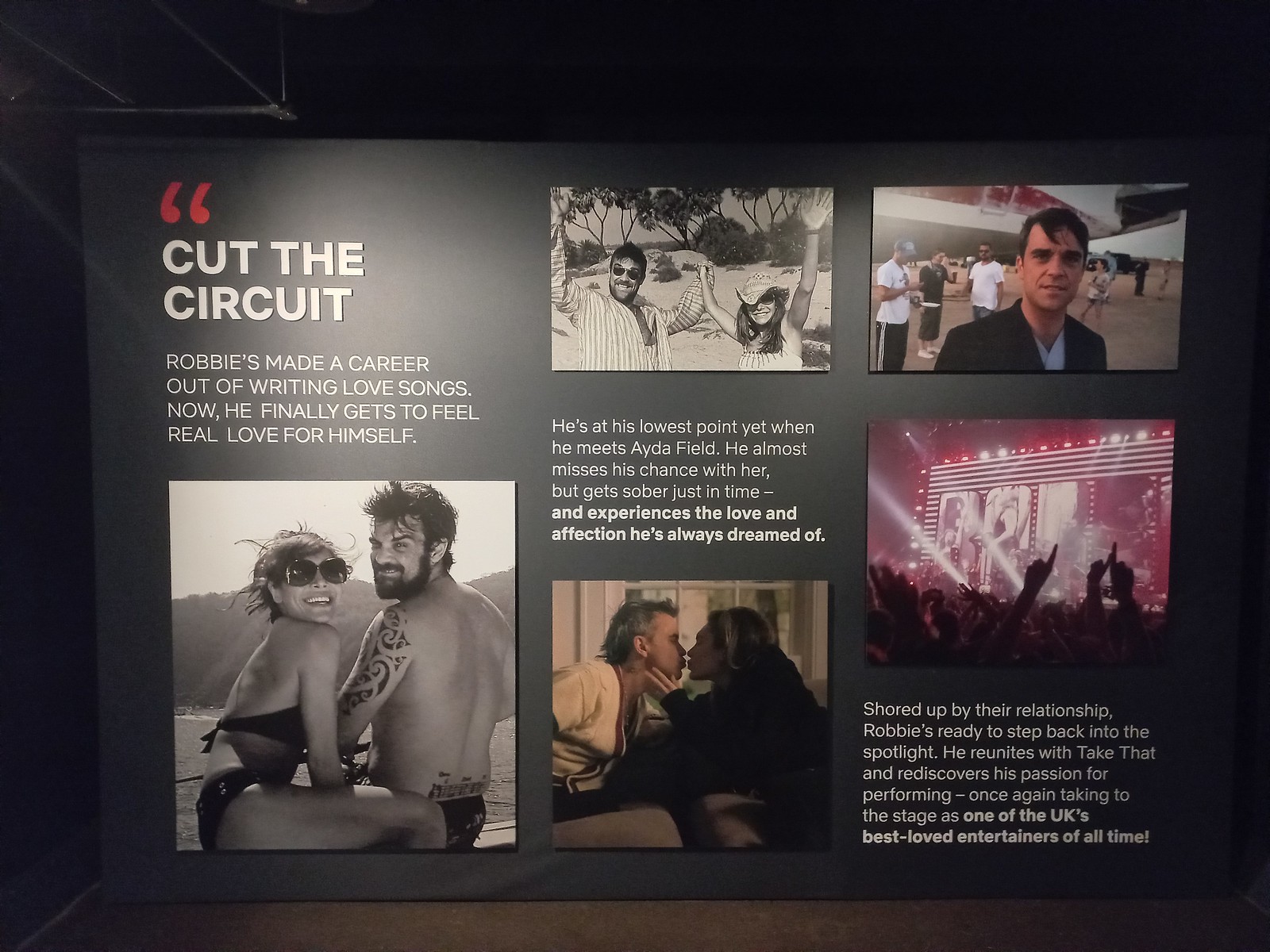This display, resembling a museum exhibit, features a series of photographs and text panels, all focused on Robbie, a man who has spent his career writing love songs and now experiences true love himself. The exhibit is organized into different panels and includes a striking title in white letters, "Cut the Circuit," positioned in the upper left corner alongside a set of red quotation marks. 

Directly below the title is a black-and-white image of a shirtless man with a tattoo sleeve on his left arm and a woman in a bikini and large sunglasses, both seated on a dock with water visible in the background. The man is turned away but looking over his left shoulder towards the camera.

In the middle column, there are two additional photos: a colored one at the bottom and a black-and-white one at the top. The black-and-white image shows a man and a woman with their arms raised in the air, while the colored photo at the bottom depicts a man and a woman kissing, the man in a white shirt and the woman in black. 

Text beside these images narrates Robbie's life transition, highlighting how he met Ada Field at a low point in his life, almost missed his chance with her, but managed to get sober just in time to experience the love he always dreamed of.

In the upper right-hand corner, there's a picture of a man in a suit with a white shirt, and towards the lower right corner, text declares that shored up by their relationship, Robbie is ready to return to the spotlight. He reunites with his band, Take That, rediscovering his passion for performing and reclaiming his status as one of the UK's most beloved entertainers. The final image shows Robbie on stage with reddish and white lights, signifying his triumphant return.